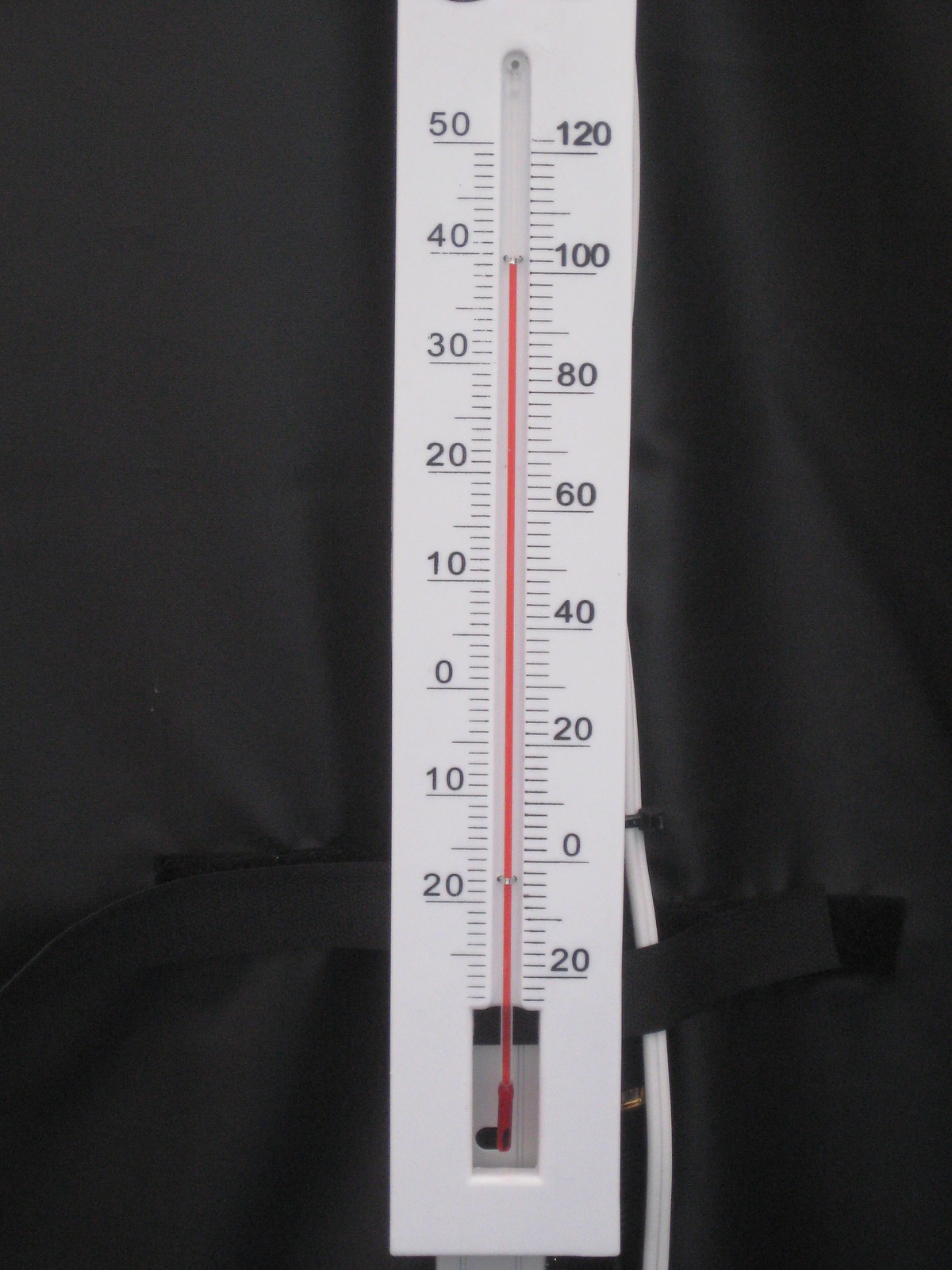The image is a close-up shot of a rectangular white thermometer with a clear gauge in the center. The thermometer features a red liquid indicator line that currently reads just above 100°F on the right and aligns with 40°C on the left. The thermometer’s temperature scale on the left side is marked in degrees Celsius, with increments of 10, ranging from -20°C to 50°C. On the right, the scale is marked in degrees Fahrenheit, also with increments of 20, ranging from -20°F to 120°F. Both the numerical and scale markings are in black.

Located on the bottom right side of the thermometer is a white tube, strapped on, suggesting that the thermometer is resting inside a black fabric case. The image is zoomed in, focusing primarily on the thermometer, which limits visibility of other surrounding details. Straps, visible on both the left and the right sides of the thermometer, secure it in place. At the very bottom of the gauge, the red indicator line is affixed with a small black attachment, ensuring accuracy in measurement.